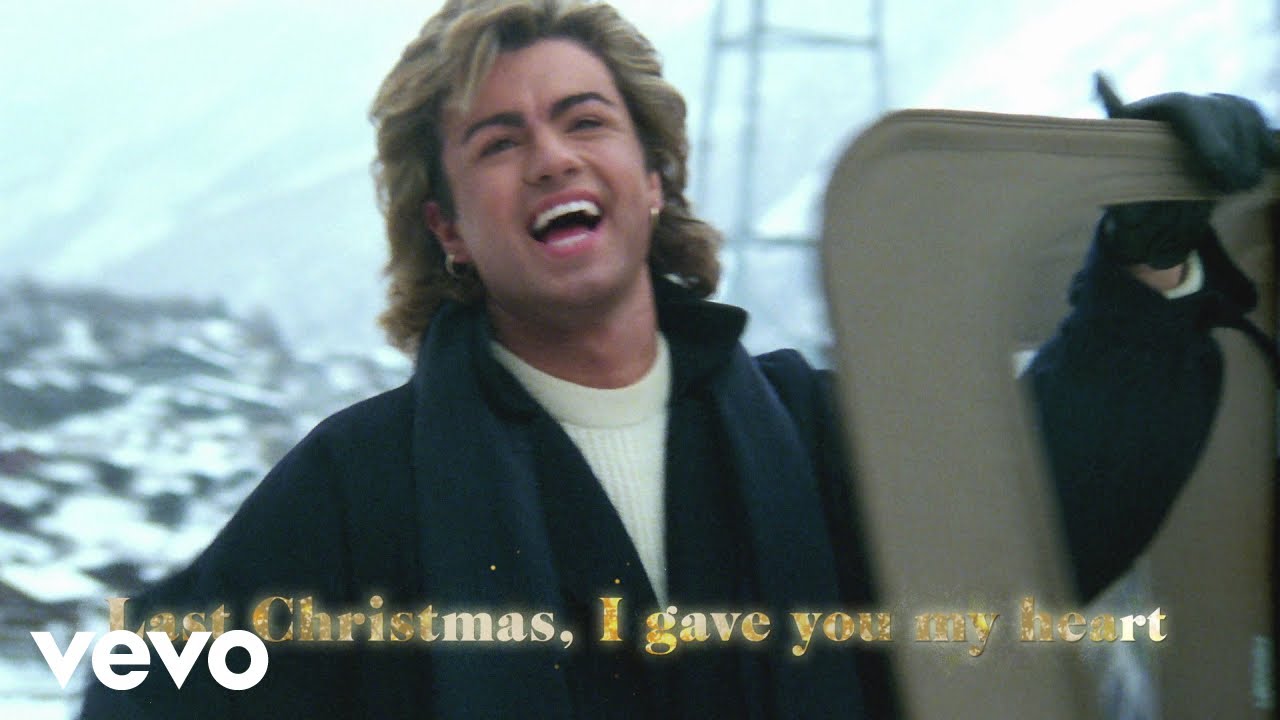The image is a horizontally aligned rectangular photo from the 1980s, featuring George Michael with his characteristic curly brown hair and thick dark eyebrows. He is opening his mouth wide, revealing his white teeth, as if singing or laughing. He sports hoop earrings in both ears. 

George is attired in a black jacket paired with a dark blue scarf and a white sweater. His right hand, clad in a black leather glove, holds up what appears to be a fabric item. There is ambiguity around what his left hand grasps, with descriptions ranging from a door to a lid, but it is primarily identified as a black object.

Below the image, in glittery gold letters, is the phrase "Last Christmas I Gave You My Heart." In the lower left corner, in bold white letters, is the word "VEVO." The background seems to display a snowy or wintry scene, with gray and white elements resembling waves, rocks, or possibly water, and the subtle outline of a mountain or tower is visible behind him. The image quality is slightly blurry.